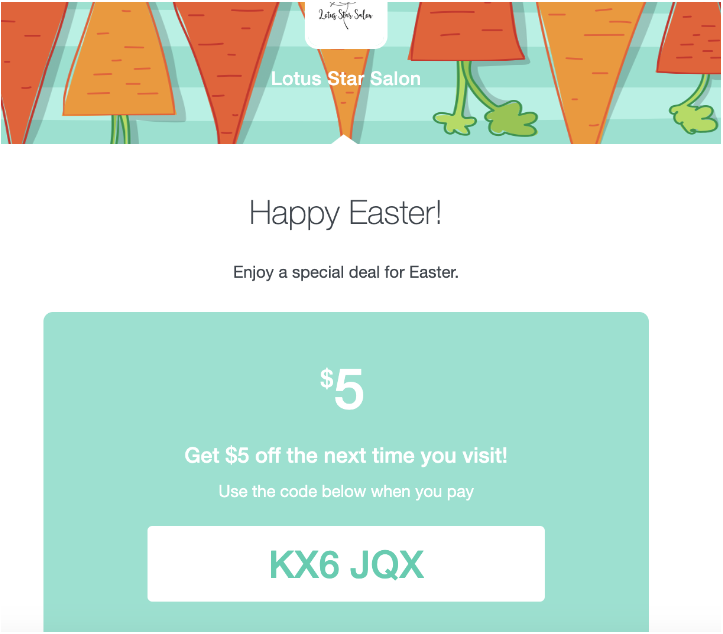The image is a promotional flyer for Lotus Star Salon, featuring a festive Easter theme. Dominating the top section is the salon’s name, "Lotus Star Salon," prominently displayed in a white and black cursive font. Surrounding the name is a vibrant assortment of carrot-like objects, each uniquely colored; some are a bright orange with green tops in a triangular shape, while others are a deeper red, also adorned with green leaves. The background behind these items is an eye-catching mix of blue stripes, adding to the Easter spirit.

Below this colorful arrangement, the flyer announces, "Happy Easter! Enjoy a special deal for Easter." Positioned on a green background is a white text box offering a $5 discount on the next visit. The instruction reads, "Use the code below when you pay," followed by the bold code "KX6JQX" within a white box accented by green coloring.

The overall layout of the flyer is predominantly white, allowing the vivid colors and details at the top to draw significant attention. The clear and concise message, adorned with festive graphics, promises an engaging and welcoming Easter promotion for all who visit the salon.